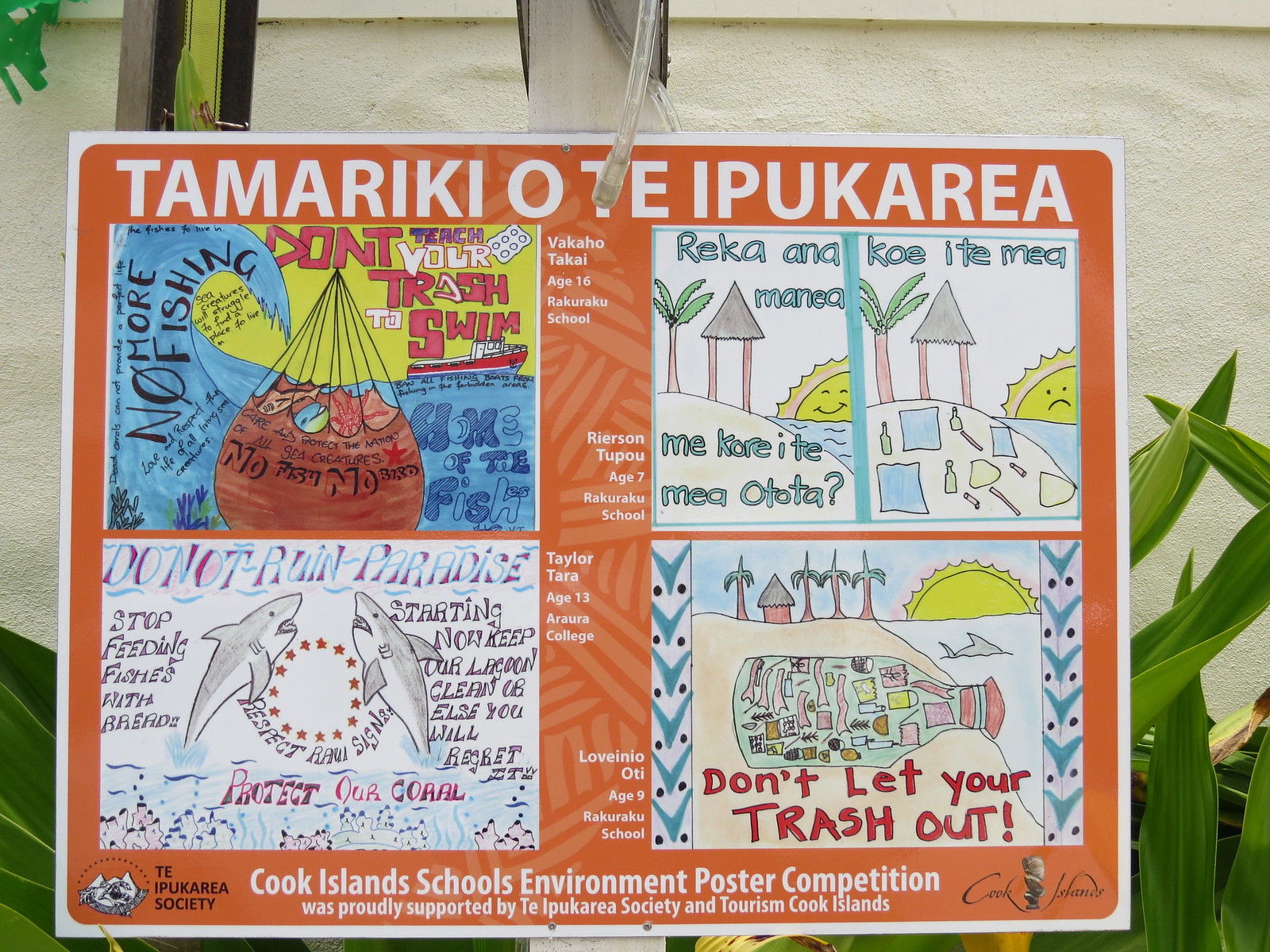This is a vibrant sign from the Cook Islands, set against an orange background with a white border. The sign features the title "Tamariki O Te Aipukaria" at the top, indicating it's part of a schools' environment poster competition, proudly supported by the Te Aipukaria Society and Tourism Cook Islands. The central theme revolves around environmental awareness, with four unique children's drawings, each occupying a corner of the sign. 

In the upper left, an illustration depicts a net catching various sea creatures, including fish and a starfish, highlighting the impact of fishing. The upper right showcases a captivating scene of the sun setting over a beach, complete with two thatched huts, palm trees, and a smiling sun, emphasizing the natural beauty of the islands. 

The lower left corner features two dynamic sharks leaping out of the ocean, surrounded by the message, "Do Not Ruin Paradise," urging viewers to protect marine life. In the lower right, there is an image of a bottle on the beach with litter inside and the cautionary slogan, "Don't Let Your Trash Out," stressing the importance of proper waste disposal. 

The entire sign is brightened with plant designs in a lighter orange shade, situated in front of a stucco building adorned with long green fronded plants, symbolizing the harmonious blend of natural beauty and cultural heritage in the Cook Islands.